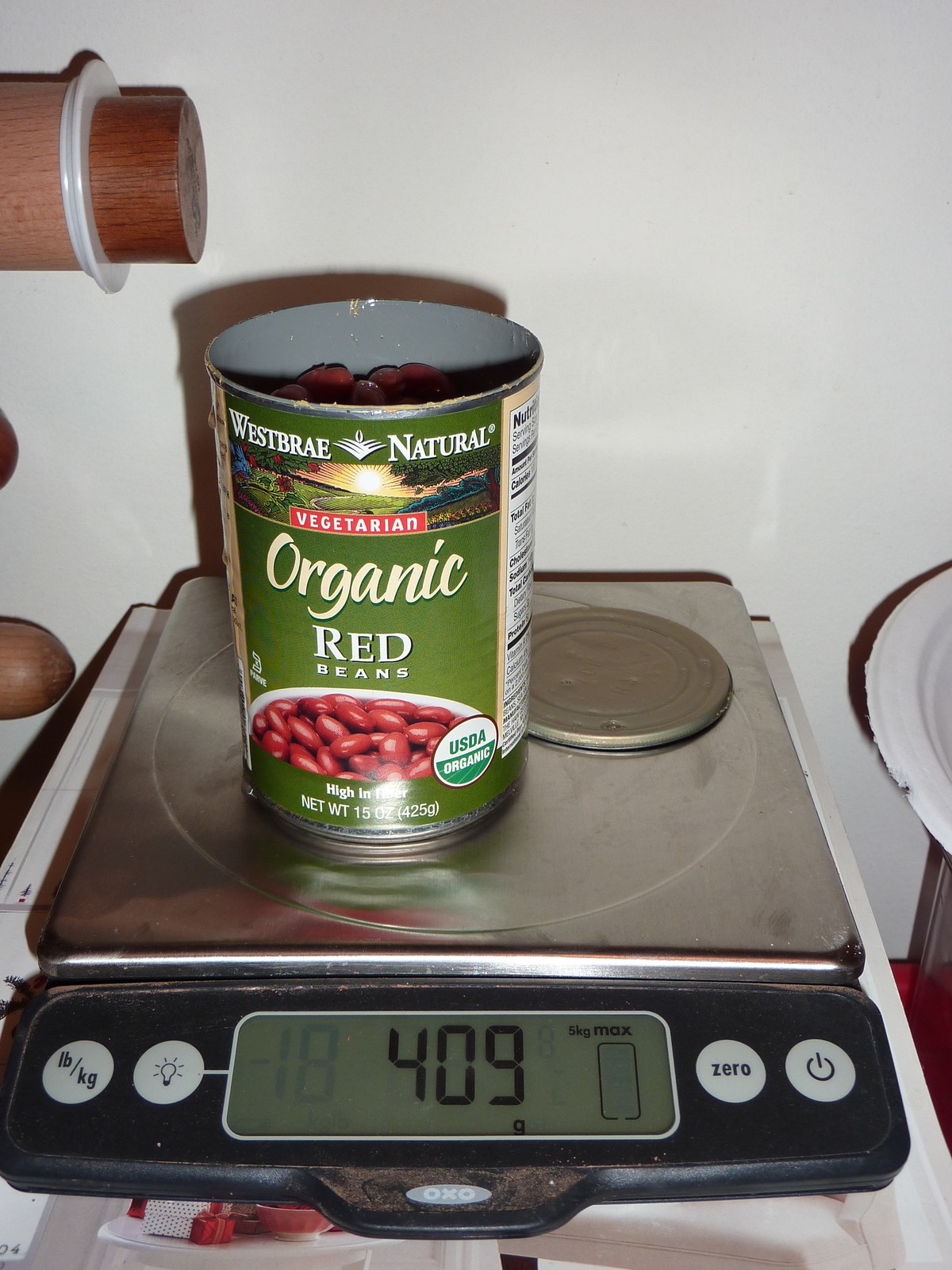The photo captures a can of Westbrae Natural Organic Red Beans prominently positioned on a metal kitchen food scale. The can features a green label with a detailed image of red beans in a white bowl. Text on the label indicates that the beans are vegetarian and organic, with a net weight of 15 ounces. The scale, which has a black front panel, displays a digital readout and is equipped with four white buttons: one for changing measurement units from pounds to kilograms, a backlight button, a zeroing out button, and a power button. The scene is set on an indeterminate surface, possibly a countertop, with a white wall in the background. Cropped in the frame are other indistinct objects, potentially including a plate on the right side, but specific details are not clearly visible.